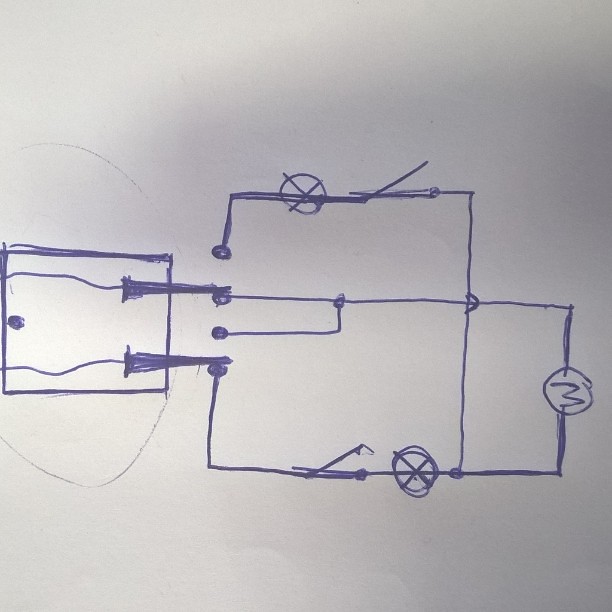This intricate schematic illustration, rendered in dark blue or black ink, presents a series of interconnected geometric shapes and symbols. Starting from the left, a square features a small circle or dot centrally placed on its left side. Radiating from this circle, wire-like lines extend upward and downward, converging towards triangular shapes that protrude outwards from the square. Adjacent to this setup is a hollow square opening, after which the original square framework continues. From the center of this extended section, two lines branch out, stretching towards the edge of the subsequent square. This next square is marked by the presence of an "M" on its right side. Additionally, it contains two "X" symbols positioned at the top and bottom of the central square. The precise arrangement and detailed connections suggest a complex diagram, possibly representing an electrical or mechanical system.